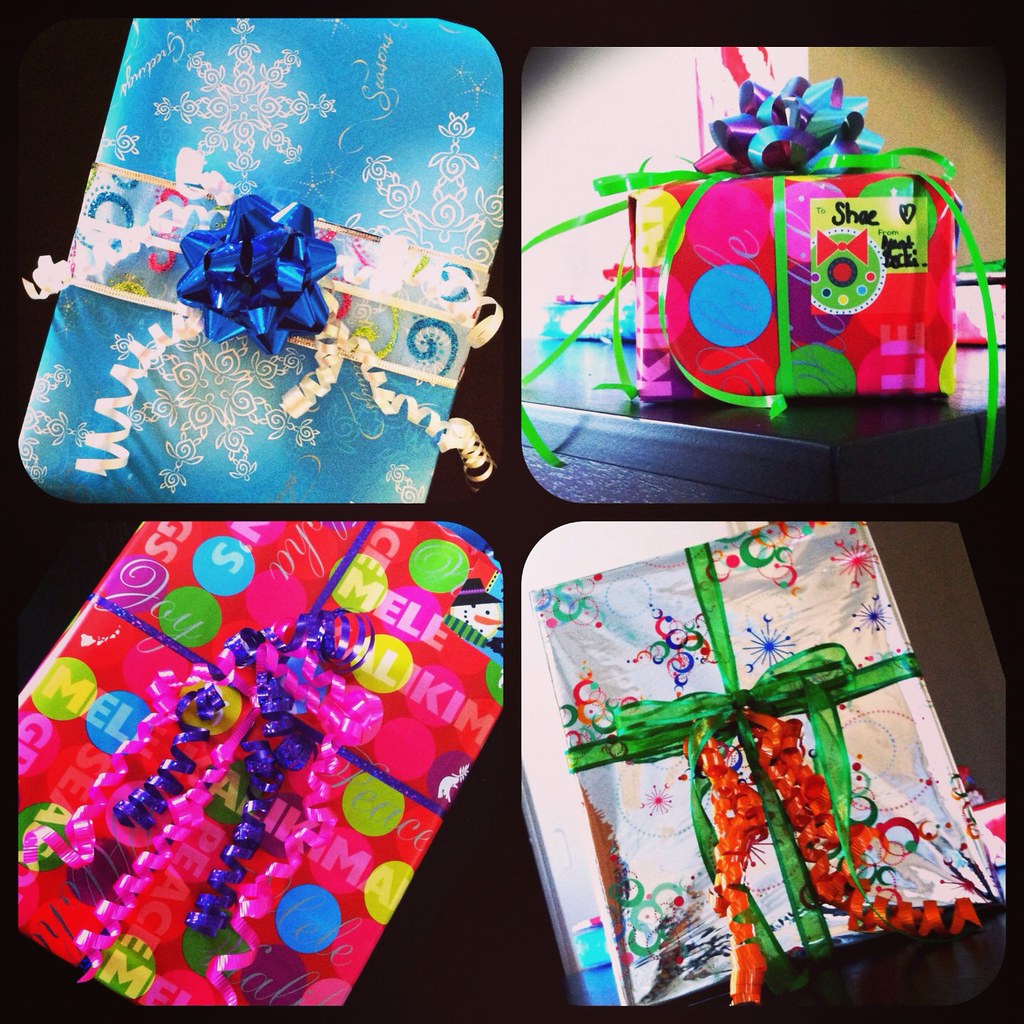The image displays a collage of four distinct pictures, each featuring a meticulously wrapped present. Starting from the upper left corner, there's a present adorned with blue snowflake wrapping paper, complemented by a matching blue bow and curled white ribbon. Moving to the upper right, the gift is wrapped in a vibrant multicolored paper showcasing various geometric shapes, primarily circles, and it’s finished with a green ribbon and a shiny blue bow. Notably, the name "Shay" is inscribed on this gift. In the bottom right, the gift stands out with its shiny silver wrapping paper, enhanced by a green ribbon and orange twirly ribbon basking in a gentle light. Lastly, in the bottom left, the present features red paper embellished with variously colored circles in green, blue, and purple, and it’s tied with both blue and pink curly ribbons. Each package is unique in its presentation and adds to the festive ambiance of the collage.